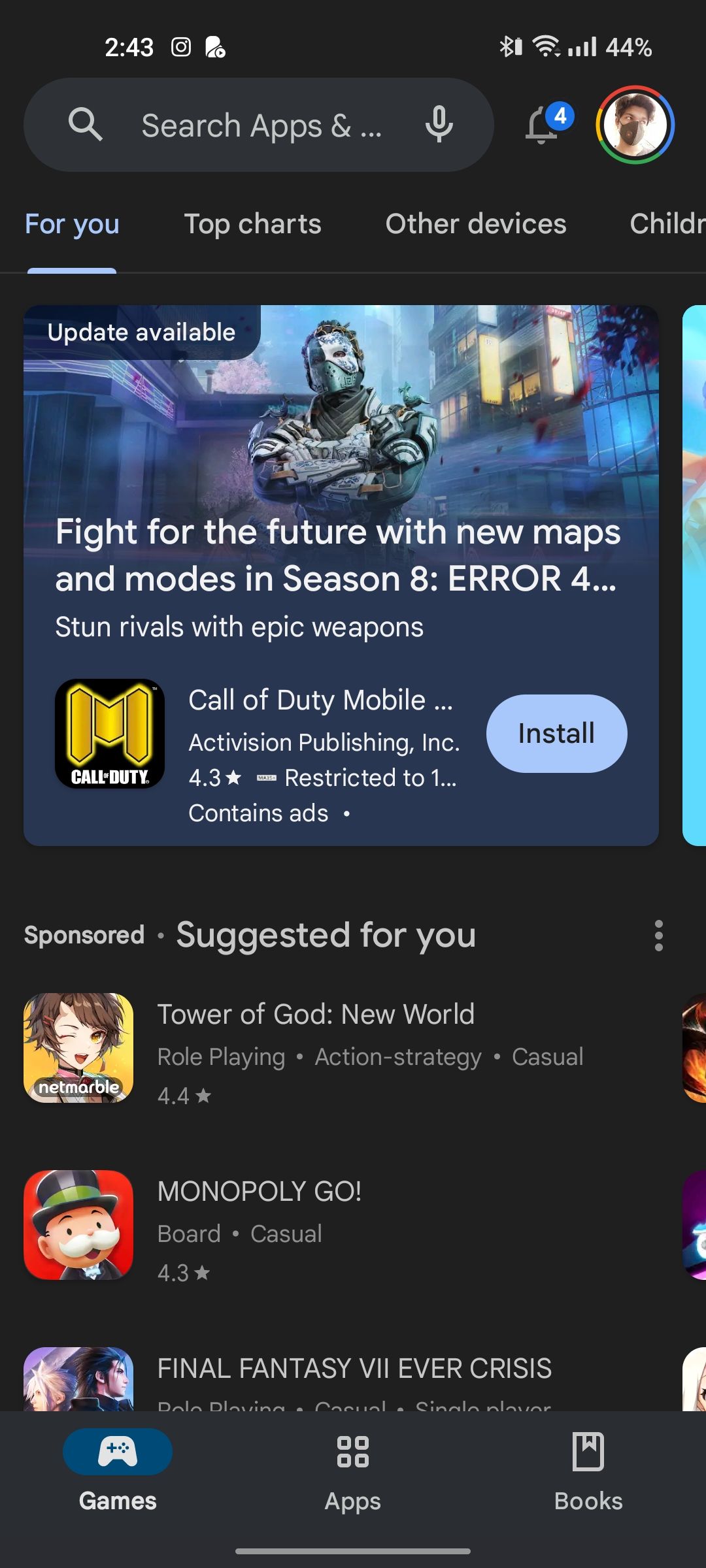### Descriptive Caption:

The image displays a smartphone screen with a predominantly black background. The top section of the screen shows the current time as 2:43, along with a battery indicator displaying four bars and a 44% battery life remaining. Just below, there's a search bar for user convenience.

In the upper part of the screen, a circular profile picture is visible, depicting a person wearing a black hat and a black mask covering their nose and mouth. Below this, a navigation menu features options such as "For You" (highlighted in blue), "Top Charts," "Other Devices," and "Update Available."

The main content area showcases an advertisement for a video game. The background of this ad features a character adorned in full grayish-blue armor, standing in a dystopian cityscape. White text overlays the image, proclaiming, "Fight for the future with new maps and modes in season eight. Stun rivals with epic weapons." It mentions the game, "Call of Duty Mobile," developed by Activision Publishing Incorporated, with an "Install" option prominently displayed in a blue circle to the right.

Below this advertisement, the screen lists several game suggestions under titles "Sponsored" and "Suggested for You." These include:
1. **Tower of God: New World**
2. **Monopoly Go** – Highlighted with a red square featuring the iconic Monopoly character with a white mustache and a black top hat.
3. **Final Fantasy Ever Crisis**